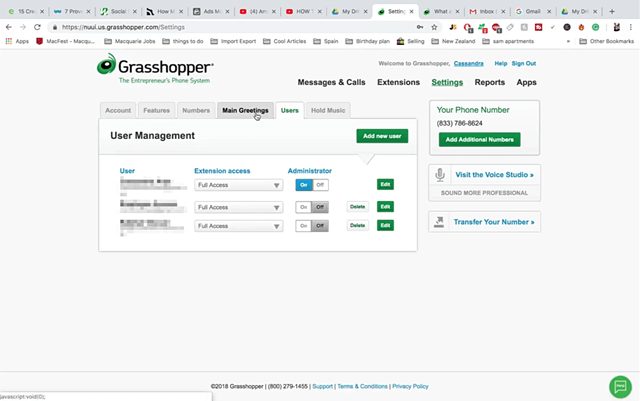The screenshot captures a web browser window with a gray banner at the top, displaying several open tabs. The tiny icons for each tab suggest that multiple YouTube tabs, some social media sites, an email inbox, and Gmail are open, totaling around 13 tabs. Additionally, there's a plus sign indicating an option to open more tabs. The active tab shows "Grasshopper," an entrepreneur's phone system, with the URL 'grasshopper.com.' 

The browser features a favorites bar and a lock icon indicating a secure connection. The Grasshopper web page is predominantly white with various interactive elements. Green buttons and blue accents highlight different sections of the interface. The navigation pane includes options like "Messages and Calls," "Extensions," and a green-highlighted "Settings" tab. Other sections shown are "Reports" and "Apps," as well as a visible phone number feature. There's an option to add additional numbers via a green button, and user management functions, including an "Add New User" button also in green.